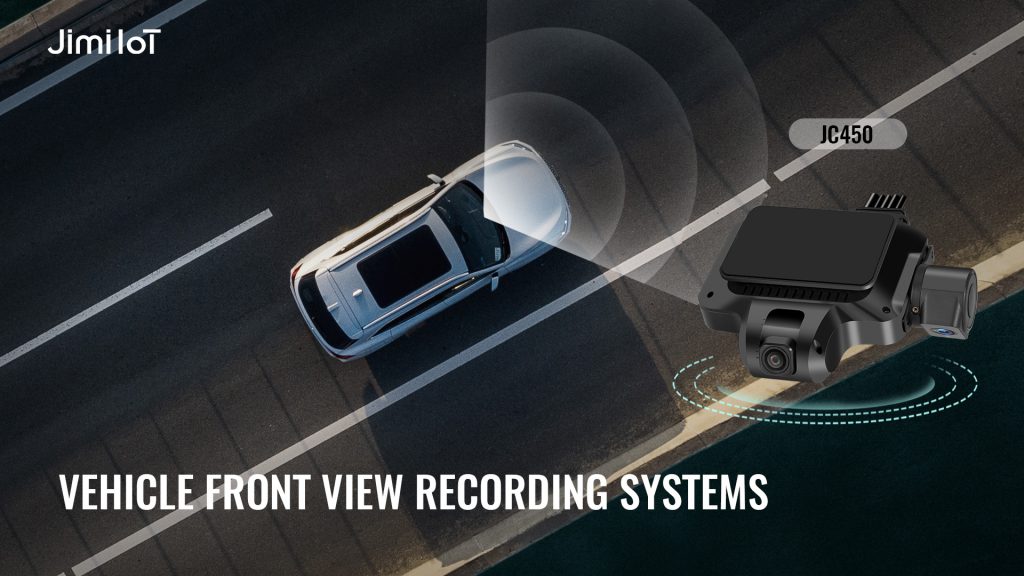The image is an illustrated, computer-generated top-down view of a small white SUV driving on a road, likely a highway. It prominently showcases a vehicle front view recording system, clearly labeled as JC450. Emitting from the SUV's dashboard is a series of white, parabolic signals, symbolizing the area being recorded by the dash cam. The top left-hand corner of the image bears the text "Jimilot" or "Jimmy Lott," possibly indicating a brand or artist. In the bottom of the image, bold white block letters declare "VEHICLE FRONT VIEW RECORDING SYSTEMS," reinforcing the depiction of the technology. Additionally, an illustrated model of the dash cam itself is positioned on the right side of the image, characterized by a gray-black device marked with the label JC450.